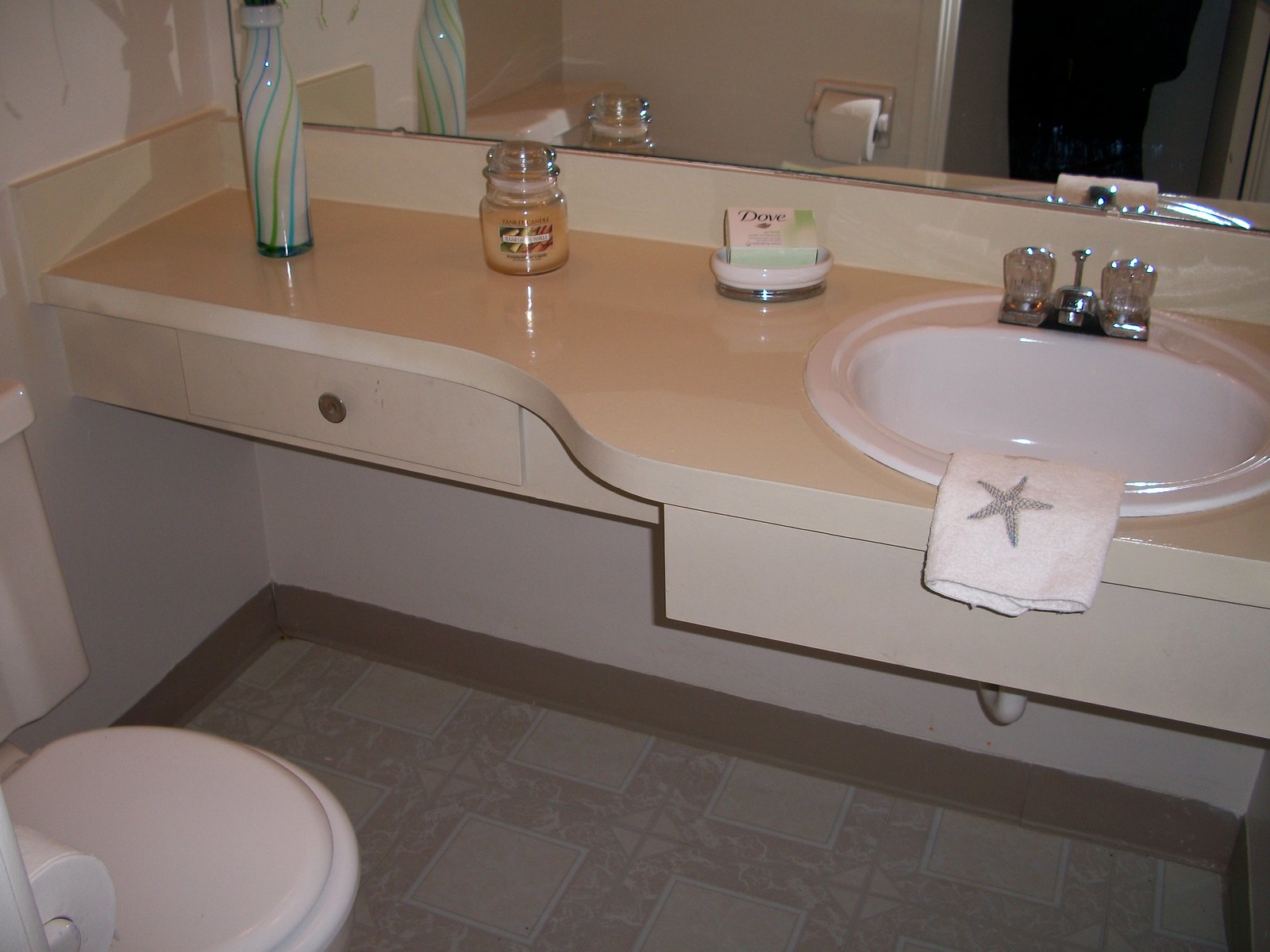The image showcases a small bathroom, primarily focusing on a light orange countertop that lacks cabinetry underneath. Instead, there is a drawer and a simple board that obscures the bottom of the sink area. The sink itself is oval-shaped, equipped with two knobs for hot and cold water. Draped over the front of the sink is a small hand towel adorned with a silver starfish pattern. 

Adjacent to the sink sits a soap dish holding an unopened bar of Dove soap. Next to the soap dish is an unlit jar candle with an orange interior, enclosed in a glass jar with a lid. Close by is a decorative glass bottle or vase, white with green and turquoise stripes spiraling upwards.

The walls of the bathroom are a tannish gray color, contributing to the room's overall understated aesthetic. In the lower right-hand corner, a white toilet and roll of toilet paper are partially visible. Above the sink, an unframed, large mirror spans the width of the wall, reflecting the room and enhancing the sense of space.